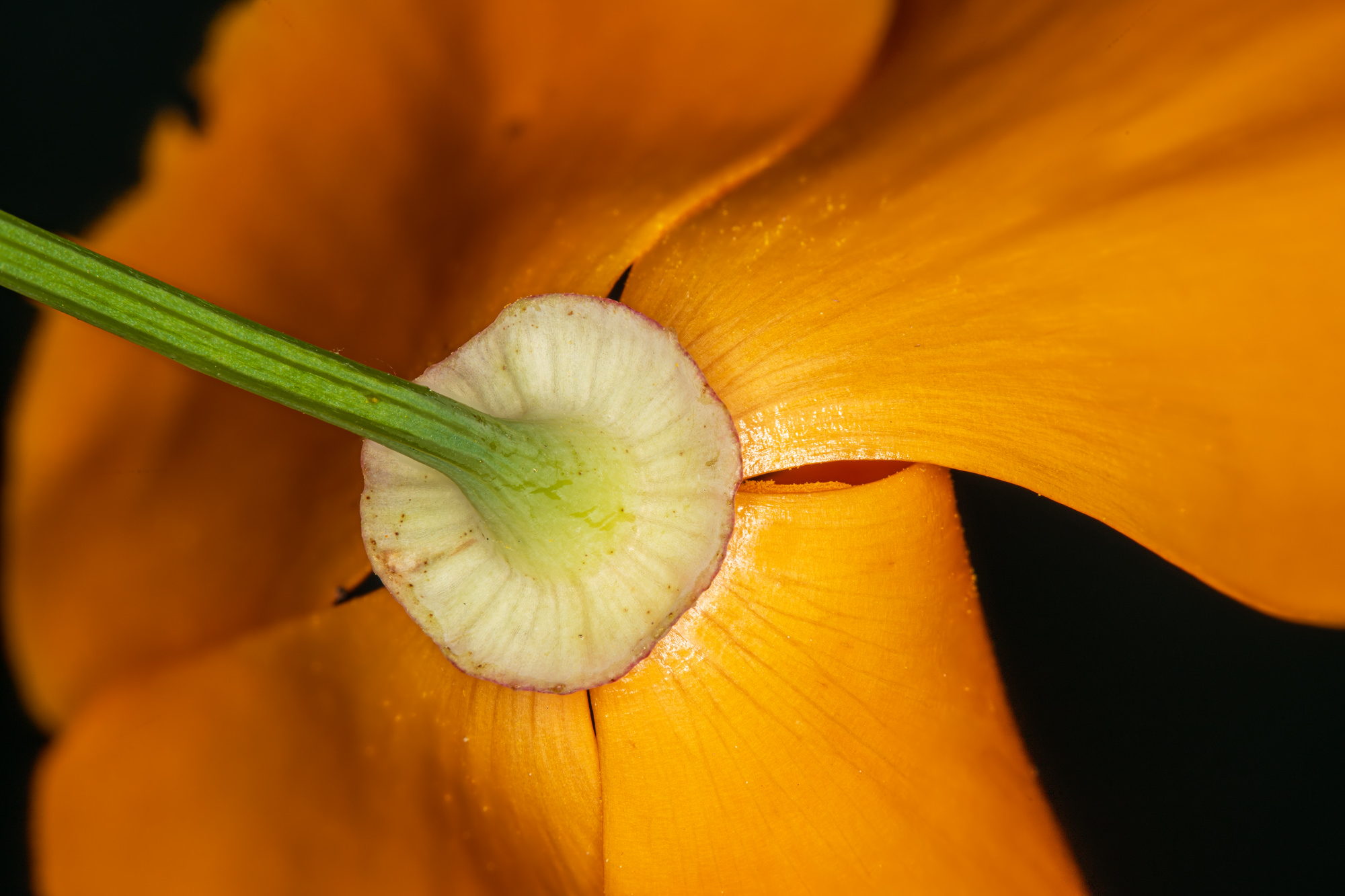This image showcases an extreme close-up of the underside of a four-petaled flower. The green stem, prominent on the left side, gradually fades into a white base where it connects to the flower. This white base fans out in a circular fashion, transitioning into petals that exhibit a rich, orange-yellow color, reminiscent of peach or pumpkin hues. The fine details of the petals' veins are clearly visible, highlighted by a glistening effect likely due to the photographer's use of a flash. The petals fan outwards from the base, creating a radiant and moist appearance. The background is a deep black, suggesting the photo was taken at night, further emphasizing the vibrant colors and intricate textures of the flower.